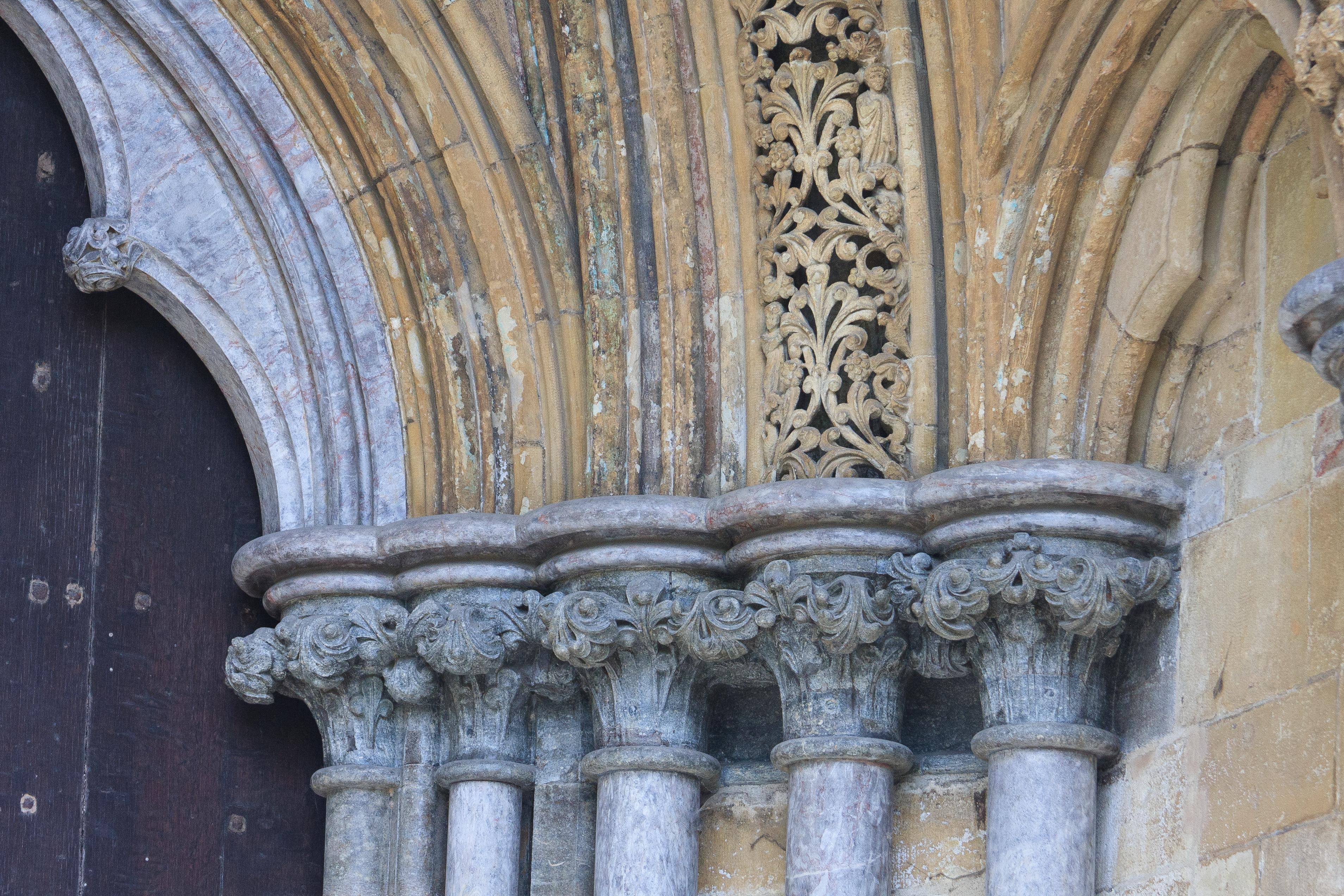This photograph depicts a section of an old stone building with intricate decorative elements, appearing reminiscent of a historic church or cathedral. The image centers on a series of five gray stone columns adorned with detailed, flowery carvings. Above these columns, the stonework transitions into a tan color, continuing the floral motifs and featuring arch-like structures that span across horizontally, some extending upwards with added design accents, including a grate with intricate patterns. To the left side of the image, there is a dark wooden door punctuated with nails, showing signs of age and wear. The overall backdrop of the scene includes a wall composed of tan and faded brown bricks, contributing to the worn and historic aura of the building.